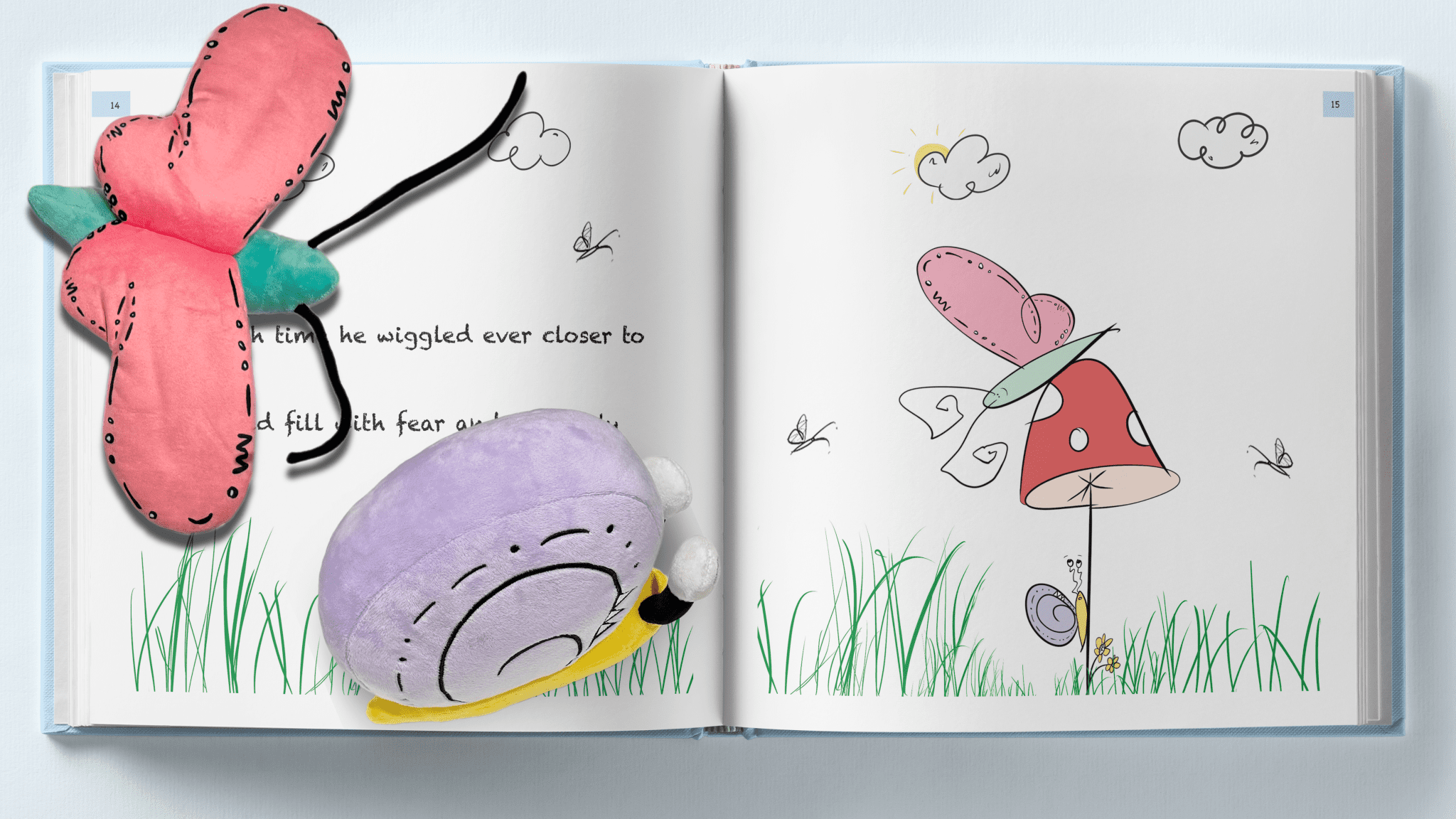This image showcases an open children's book displayed on a white table, taking up the majority of the screen. The book is open to pages 14 and 15, with an engaging blend of 2D illustrations and 3D plush toys that make the scene come to life. On page 14, the left side, there are plush toys: a large butterfly with a green body and pink wings, and a tiny snail with a purple shell and yellow body. These plush toys are situated on top of crude, childlike drawings of grass, clouds, and black butterflies, partially obscuring the text. Readable text includes phrases like "he wiggled ever closer to" and "filled with fear."

On page 15, the right side, the illustrations mirror the plush toys with a red mushroom with white spots as the focal point. Perched on top of the mushroom is a butterfly with an orange wing and green body, while a small snail is crawling up the mushroom's stem. The scene is completed with more crudely drawn grass, clouds, and butterflies, creating a cohesive and charming visual narrative that delights and engages young readers. The combination of tangible plush toys and vivid illustrations suggests an interactive element to the book, appealing to children's tactile and visual senses.